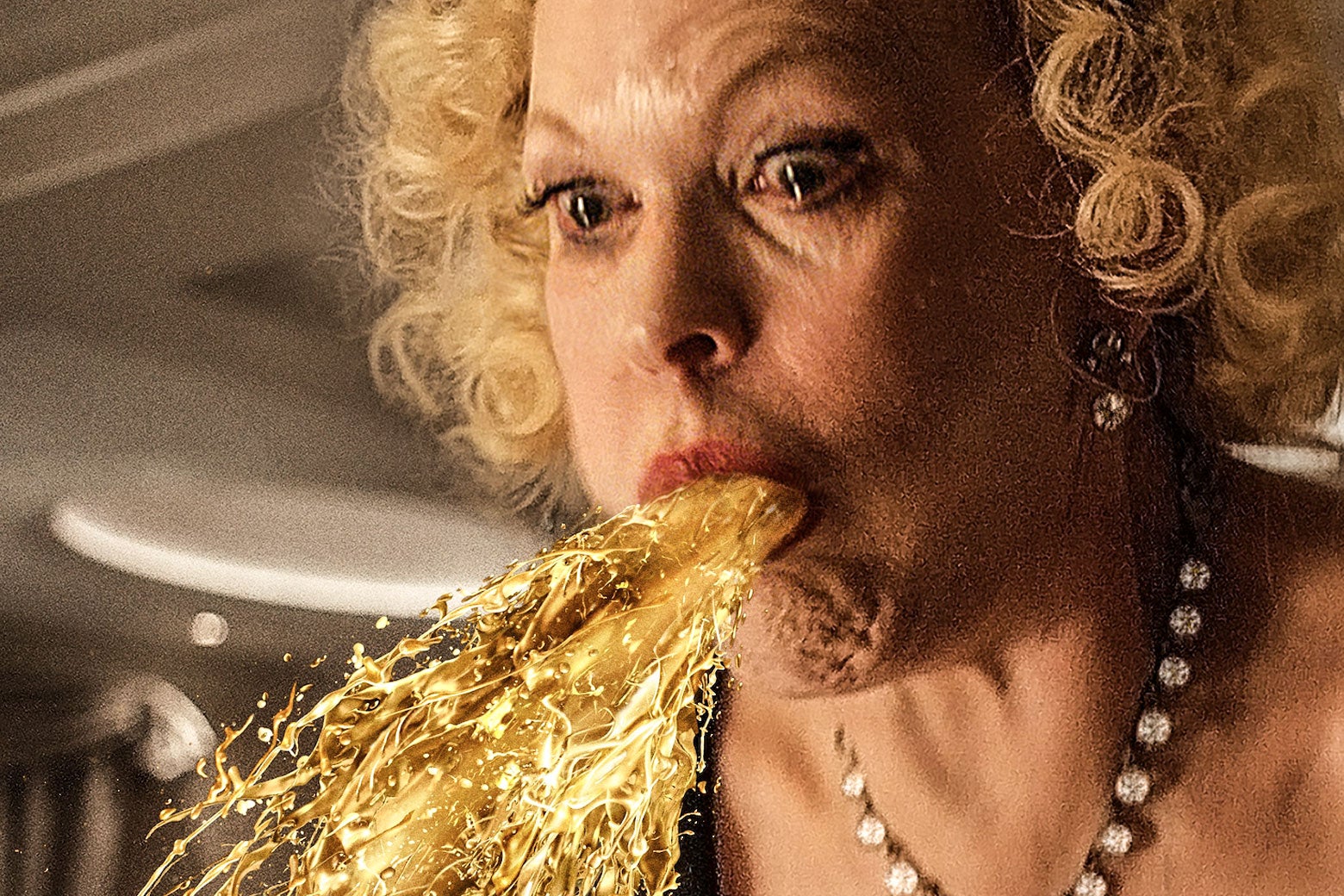The image portrays a middle-aged woman with curly blonde hair, adorned with a jewel-studded necklace and a noticeable earring in her right ear. Her facial expression conveys discomfort or disgust as she appears to be vomiting a golden, liquid-like substance that seems altered, likely through Photoshop, given its unusually bright and detailed appearance. The liquid is depicted flowing towards the bottom left of the image. Behind her, there is a blurred white wall and a faint, indistinct dot on the left side. The collar of her shirt does not reach her neckline, revealing a bit of her collarbone.